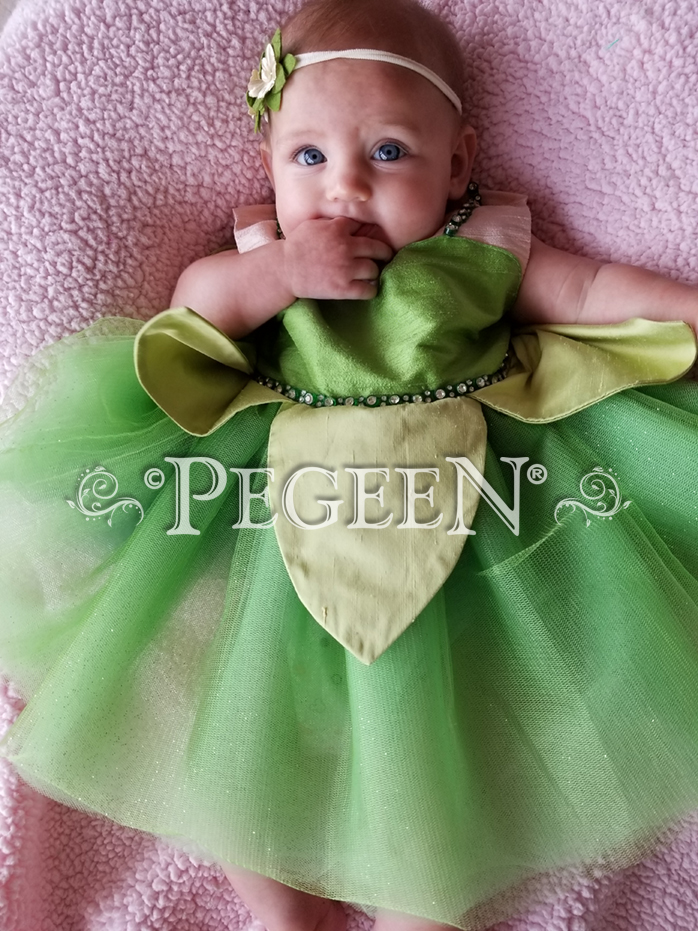In the image, a baby girl is laying on a pink fuzzy blanket, taking up a large portion of the frame and positioned directly in its center. The baby has soft brown hair, big blue eyes, chubby cheeks, and light skin. She is wearing a sleeveless green dress with a pink accent around the shoulders, a thin bedazzled black belt at the waist, and a green tutu-like skirt adorned with lighter green leaf decorations. On her head, she has a ribbon headband featuring a green and white flower on the left side. Her left arm is outstretched on the blanket, while her right arm is bent at the elbow with her finger in her mouth. Overlaid text near the center of the image reads "Pete Peggin," alongside decorative leafy scroll images, indicating a possible brand name or advertisement. The colors in the scene include various shades of pink, green, yellow, white, brown, and blue, creating a vibrant and heartwarming portrayal of the baby in a cozy, resting setting.